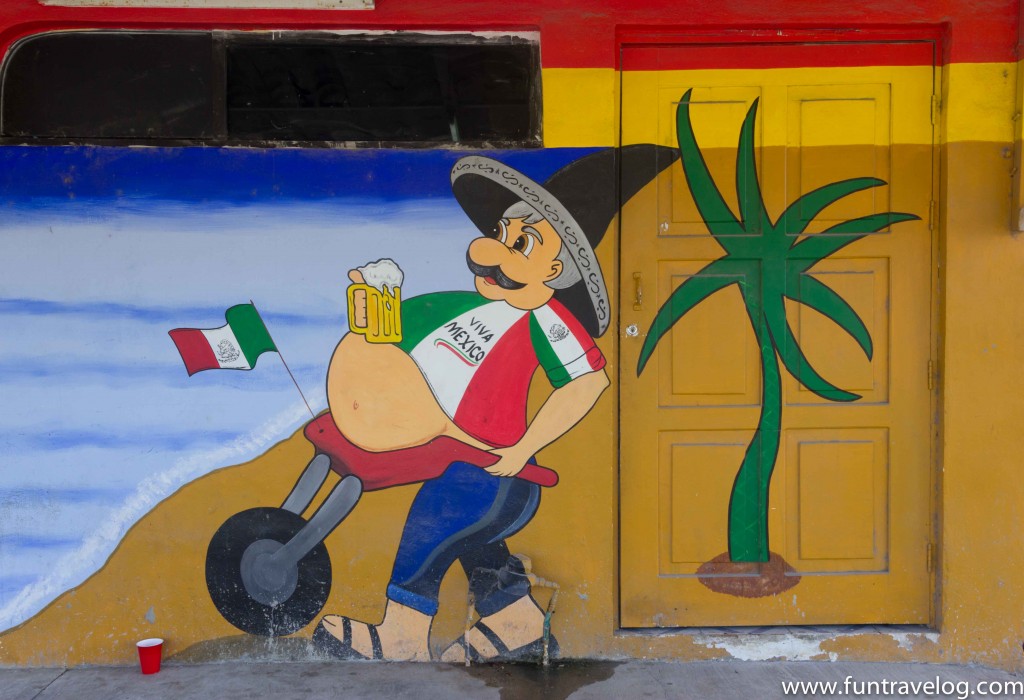This is a cartoon image of a Hispanic man with a large belly, depicted as a mural painted on the front of a building. The man is wearing a black sombrero and has gray hair and a long mustache. His shirt, in the colors of the Mexican flag (red, white, and green), features the words "Viva Mexico" across the chest. He is pushing a red wheelbarrow with a black wheel, and his large belly hangs over it. In his right hand, he holds a yellow mug of foaming beer. The wheelbarrow has a green, white, and red flag protruding from its side. The man is walking along a sidewalk in black sandals, and to his right is an old-looking door painted in red and yellow with a palm tree on it. The building itself is mainly painted in orange and yellow-orange colors, with thin horizontal strips of bright yellow and red at the top. In the lower right-hand corner of the mural, the website "www.funtravellog.com" is printed in white.